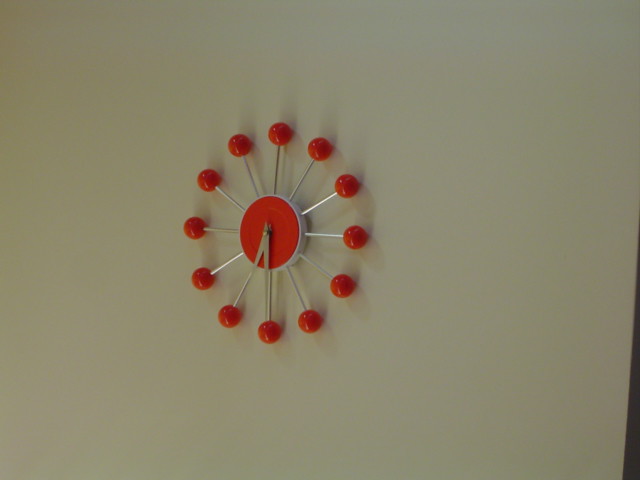A light olive green wall serves as the backdrop for a striking and unconventional clock. The clock features a red centerpiece from which silver rods extend outward, each ending in a small red ball. These balls, uniformly arranged in a circular fashion, denote the hours. The minute and hour hands, also silver, indicate a time of approximately 7:30. The clock's symmetrical design, accentuated by the consistent placement of the red balls at the ends of the rods, creates a visually engaging and artistic display. While it may not suit everyone's taste, the inventive concept and balanced aesthetic certainly make it a noteworthy piece.